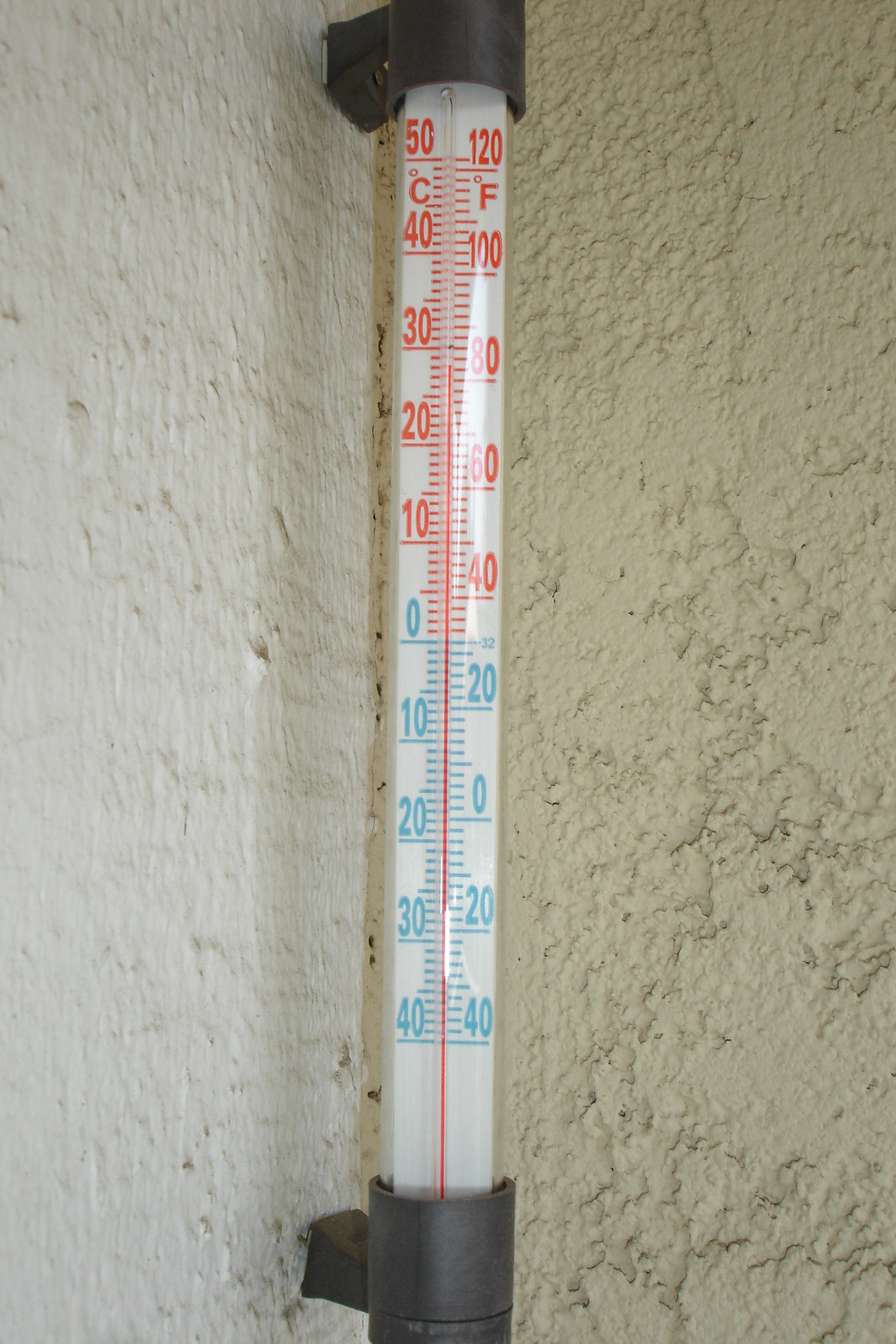The photograph depicts an exterior wall of a house or building, painted in an off-white color and featuring a highly textured stucco finish. Mounted to this wall with black plastic brackets is a classic glass thermometer containing mercury. The thermometer displays temperature readings in both Celsius and Fahrenheit. On the left side, the Celsius scale ranges from 50 down to -40 degrees, while on the right side, the Fahrenheit scale ranges from 120 down to -40 degrees. The current temperature indicated by the mercury is approximately 28 degrees Celsius (82 degrees Fahrenheit).